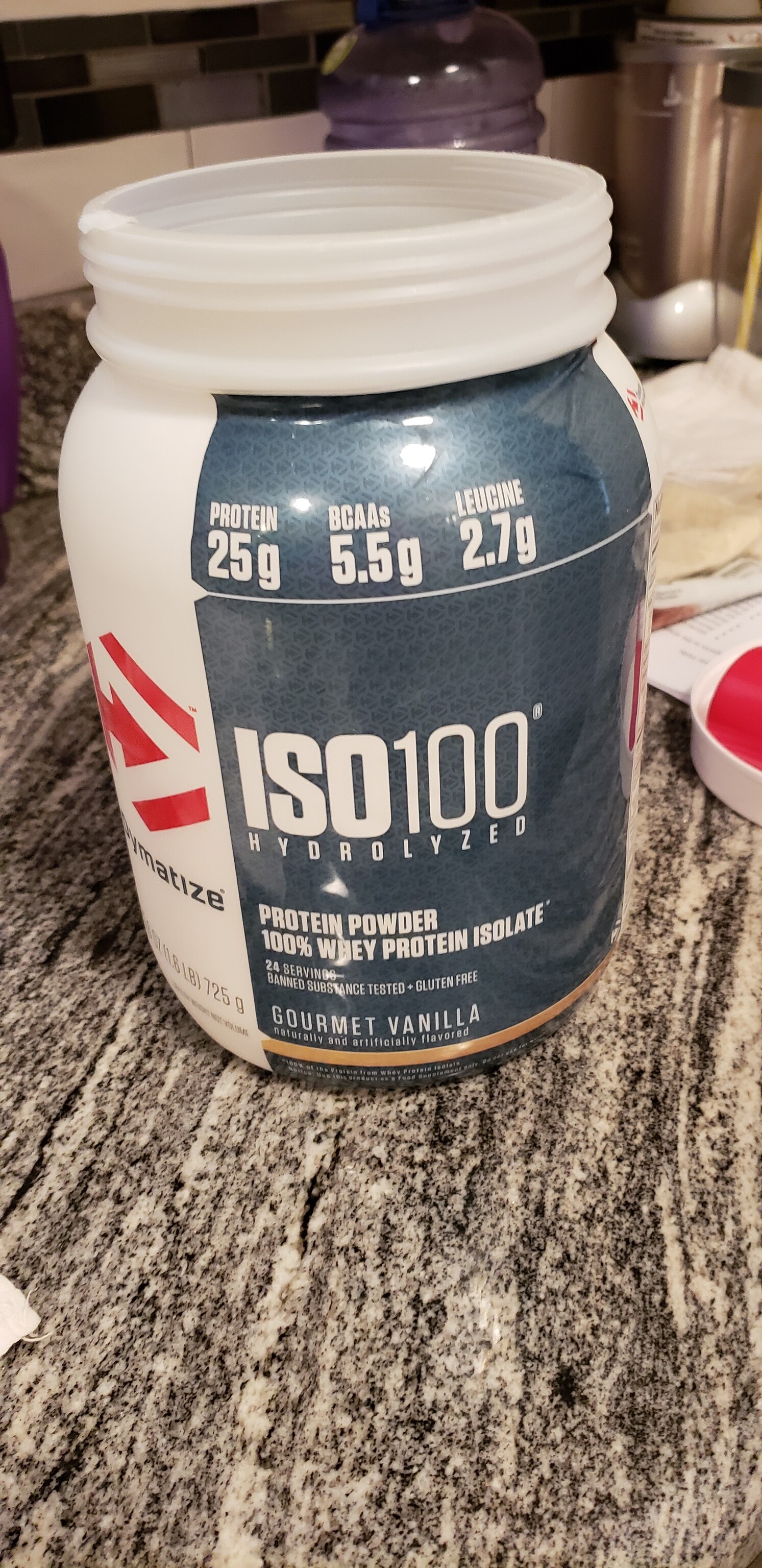This close-up photograph captures the upper section of a kitchen countertop, distinguished by its black and beige granite or marble-like surface. Dominating the center of the image is a plastic container of ISO 100 protein powder in gourmet vanilla flavor. The brand name "ISO 100" is prominently displayed in bold letters on the container, with "hydrolyzed" in smaller white text beneath it. Additional detailed descriptions and nutritional information, including the highlight of 25 grams of protein per serving, adorn the top of the label.

To the right side of the container, the lid is casually placed, resting on the corner of what appears to be a notepad or a small stack of papers. The background features an assortment of small household appliances, contributing to the everyday kitchen environment depicted in the scene.